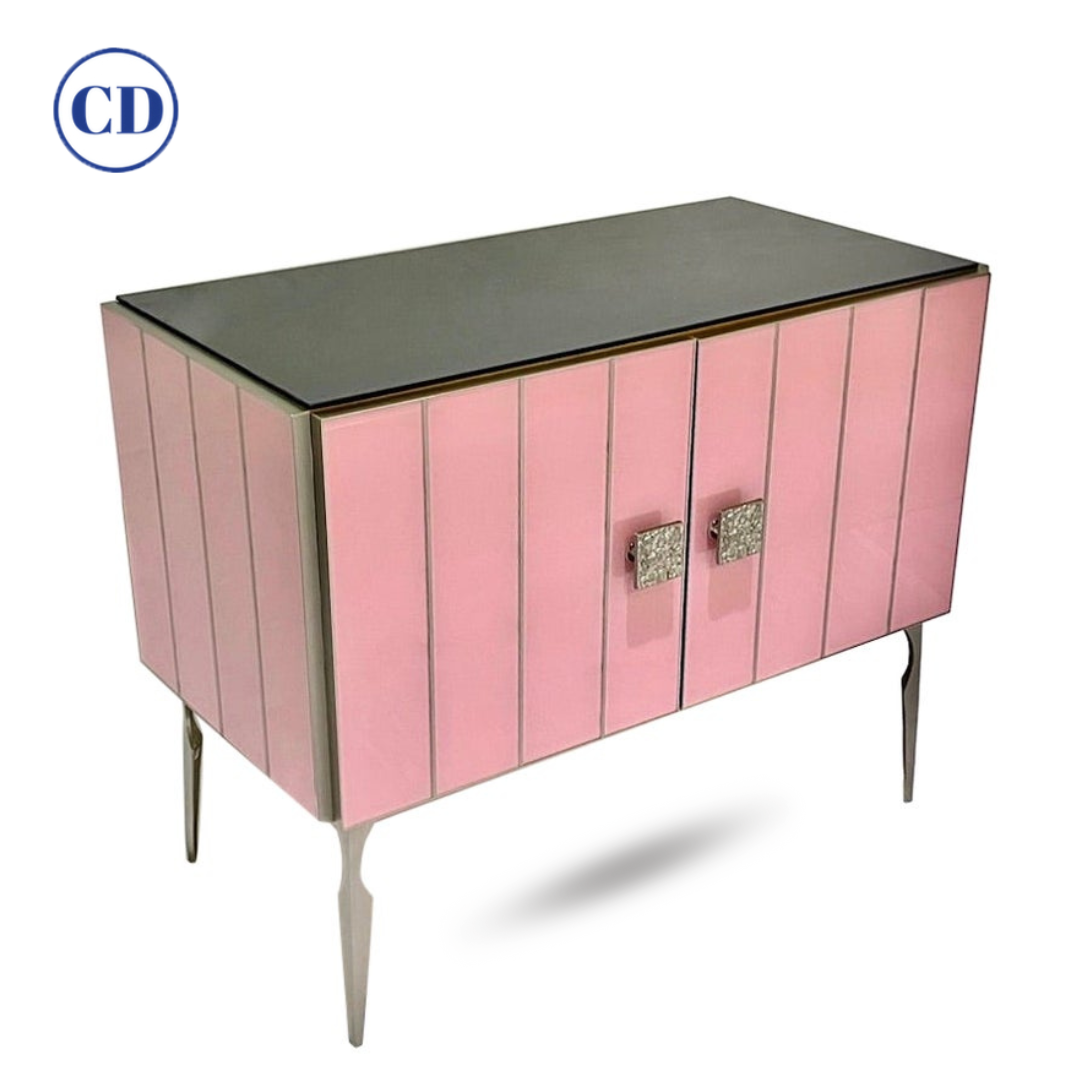This image depicts a small, vintage-style piece of furniture, likely a side table or a small dresser, with distinct decorative elements. The furniture is primarily made out of wood and features a top surface that is black. The front and sides are adorned with vertically aligned pink slats. It has thin, tapered legs, three of which are visible due to the angle of the photograph, that appear delicate and might suggest limited weight-bearing capacity.

At the front, there are two square handles that stand side by side, possibly made of cork or wood, with a textured, glittery appearance, casting small shadows beneath them. These handles suggest that the front panel opens outward, though the exact mechanism is unclear from the image. Positioned on the legs, the furniture creates a slight shadow beneath it. 

In the top left corner of the image is a circular blue logo containing the initials "C" and "D." The rest of the background is plain white, emphasizing the contrast and clean design of the piece of furniture. The furniture appears to be angled so that the left side faces slightly towards the viewer, enhancing the visual depth of the composition.